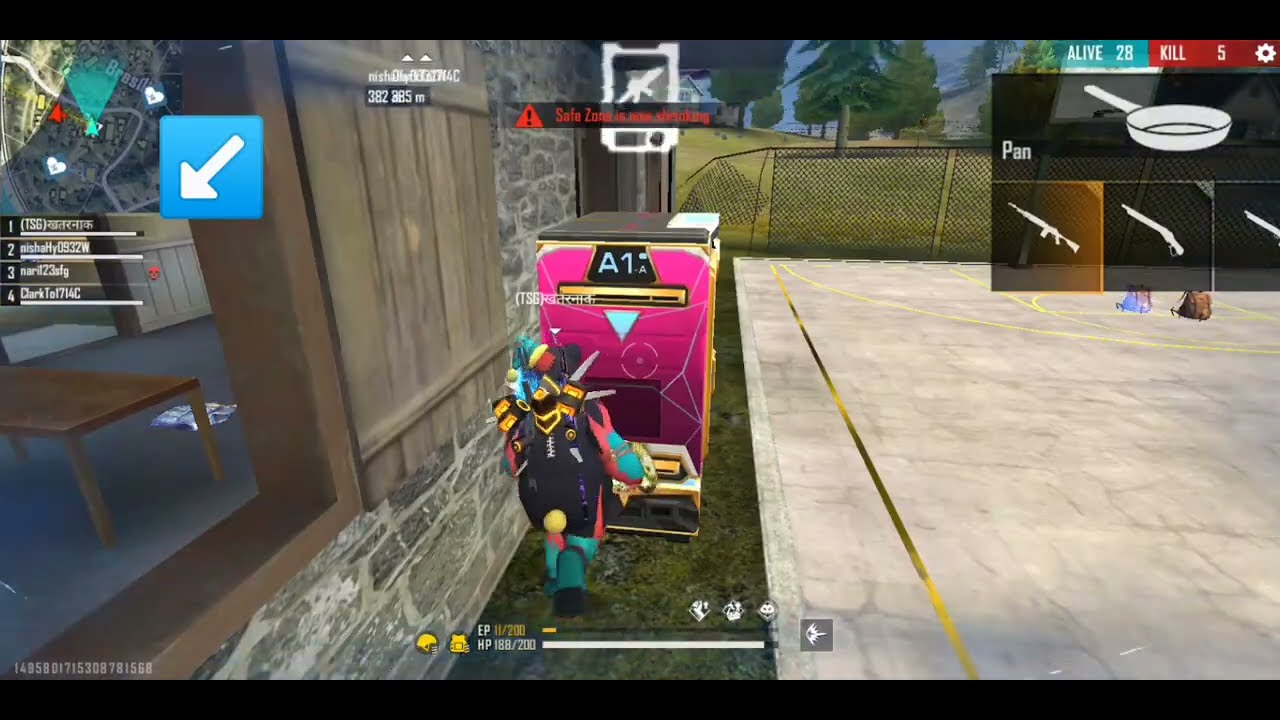The image is a screenshot from a video game, possibly PlayerUnknown's Battlegrounds or a similar battle royale game. The scene is set outdoors next to a gray stone building with a brown wooden shutter. The protagonist, who is the main character controlled by the player, stands out prominently. This character has a black spiky shoulder setup, a yellow and black striped neck gear, a red long-sleeved outfit, and blue legs, with an additional black shield and green legs visible. 

He is interacting with or facing a pink, prism-like box labeled "A1," which features a brown top. This might be a vending machine or some other type of interactive object, as the context implies potential actions like pulling or baking. Various status indicators and game UI elements are visible, including health points (HP) showing 188 out of 200 and additional bars labeled EP.

The environment includes a basketball court with cracked concrete and yellow lines, right next to grassy terrain and a forest with broken fencing. In the game's HUD, the top right corner displays "Alive 28" and "Kill 5," suggesting survival statistics. A frying pan icon and several weapons are also shown, accompanied by the word "pan." Additional interface elements include a mini-map in the top left corner, names of other players, and notifications such as "the safe zone is now shrinking." The backdrop features a mixture of gray stone, green grass, and trees, encapsulating a dynamic open-world environment.